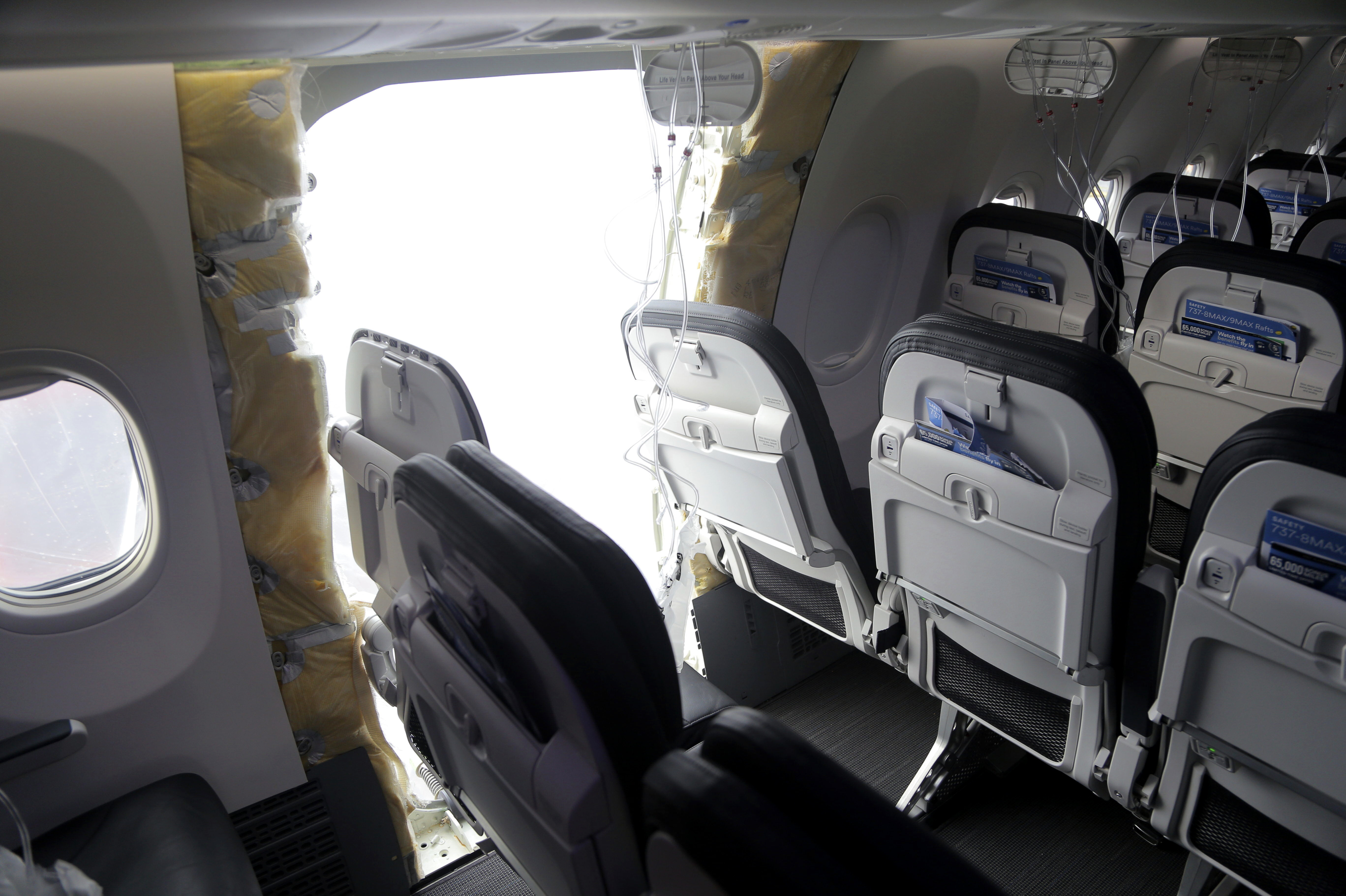This image depicts the interior view of an airplane, focusing on an open emergency door that reveals yellow-orange insulation wrapped in plastic. The outside scene through the door frame appears as a featureless, gray-white expanse, suggesting dense clouds or mist. The cabin is notably empty of passengers, with dark black and gray leather seats arranged in rows. Each seat back includes a blue and a black pamphlet, possibly in-flight magazines, stored in their pockets. Clear, translucent wires, presumably from the overhead safety masks, dangle in front of each seat. The seat tray tables are light gray, providing a contrast to the darker seating. The aircraft, despite the missing door, appears to be in good condition. The floor inside the plane is black, complementing the overall color scheme of the interior.